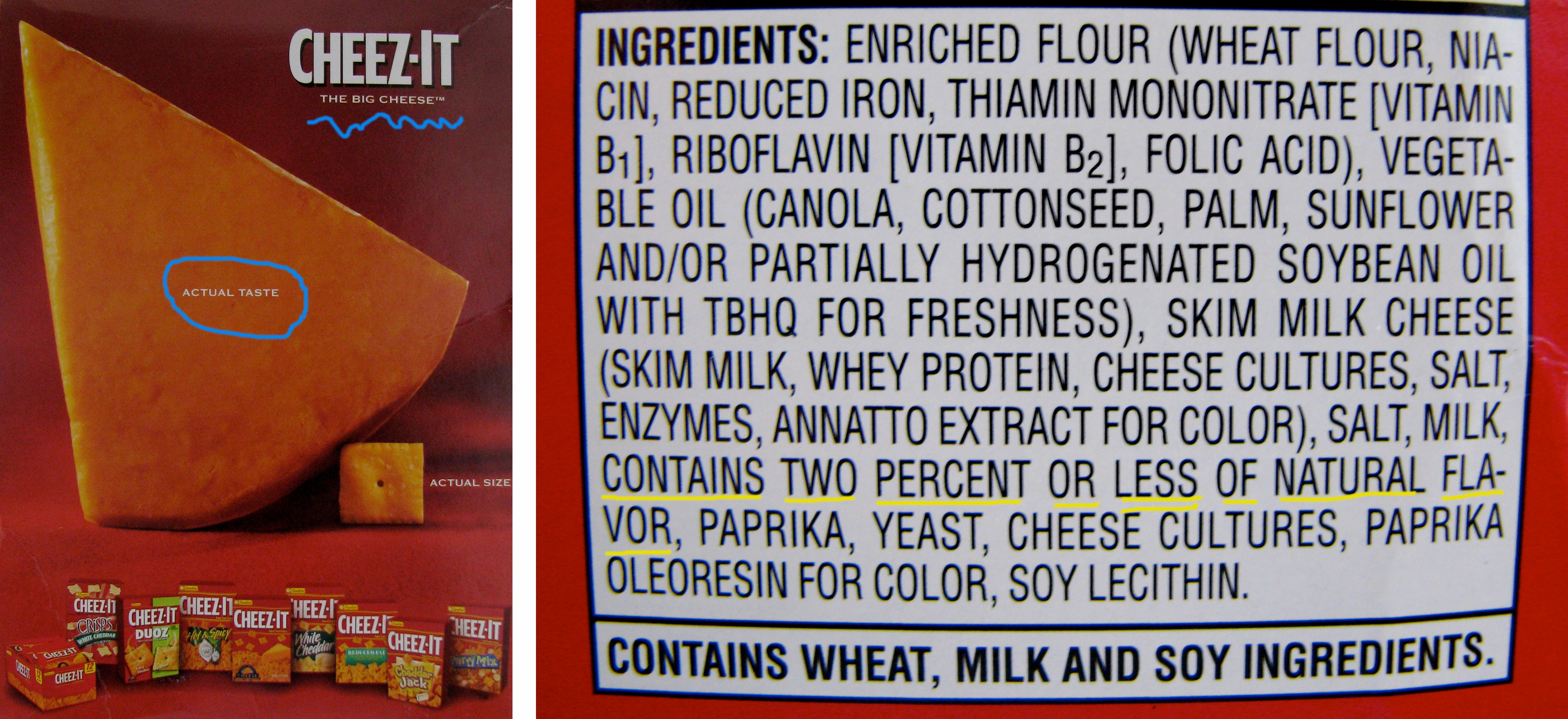This image prominently features a Cheez-It box, divided into two distinct sections. On the right-hand side, occupying about two-thirds of the frame, is a close-up view showcasing the ingredients list against a red background. The word "INGREDIENTS" is in bold, followed by a detailed list in capitalized letters: enriched flour (wheat flour, niacin, reduced iron, thiamine mononitrate [Vitamin B1], riboflavin [Vitamin B2], folic acid), vegetable oil (canola, cottonseed, palm, sunflower, and/or partially hydrogenated soybean oil with TBHQ for freshness), skim milk, cheese (skim milk, whey protein, cheese cultures, salt, enzymes, annatto extract for color), salt, along with less than 2% of natural flavor (underlined in yellow), paprika, yeast, cheese cultures, paprika oleoresin for color, and soy lecithin. At the end of the ingredients list, it notes in capital letters that the product "CONTAINS WHEAT, MILK, AND SOY INGREDIENTS."

The left-hand side, making up approximately one-third of the screen, features a vibrant advertisement for Cheez-Its. At the top, the word "Cheez-It" is prominently displayed, followed by the tagline "The Big Cheese" in small white letters. This portion of the image has a red background, accented by a blue squiggly line under the tagline. Below is a large, triangular wedge of cheese with the phrase "ACTUAL TASTE" in white letters inside a blue circle. Adjacent to this is a small Cheez-It cracker labeled "ACTUAL SIZE." At the bottom of this section, there are nine different variations of Cheez-It boxes neatly arranged: Duoz, Hot & Spicy, White Cheddar, Cheddar Jack, Party Mix, Reduced Fat (placed between White Cheddar and Cheddar Jack), and two indistinguishable varieties, with the far-left one being unclear.